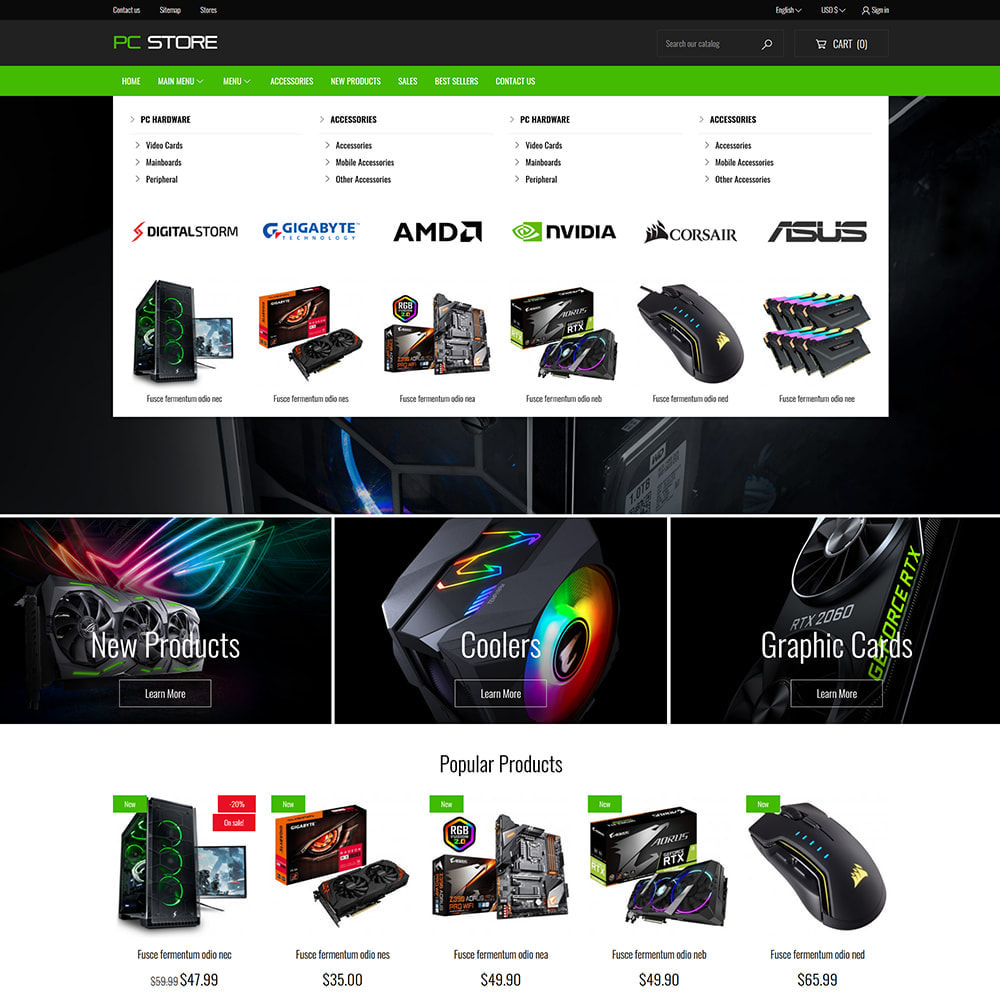This image is a screenshot of a computer interface displaying an online PC store. At the very top, there are several small, unreadable links and drop-down menus. Directly below is the store's name: "PC Store," with "PC" highlighted in green and "Store" in white against a black background. On the right side of this header, there’s a search bar followed by a cart icon.

The main navigation menu below includes options such as Home, Main Menu, Menu, Accessories, New Products, Sales, Best Sellers, and Contact Us. Further down, there is another set of drop-down menus categorized under PC Hardware which expands into Video Cards, Main Boards, and Peripheral options. Additionally, there are sections for Accessories including Mobile Accessories and Other Accessories, each with further sub-categories.

Below these menus, the interface showcases a variety of product images and company logos. Near the bottom, users can see three specific categories: New Products, Coolers, and Graphics Cards. Following these categories, the page features advertisements for different products under the section titled Popular Products, all equipped with clickable links that allow users to view more details about each item.